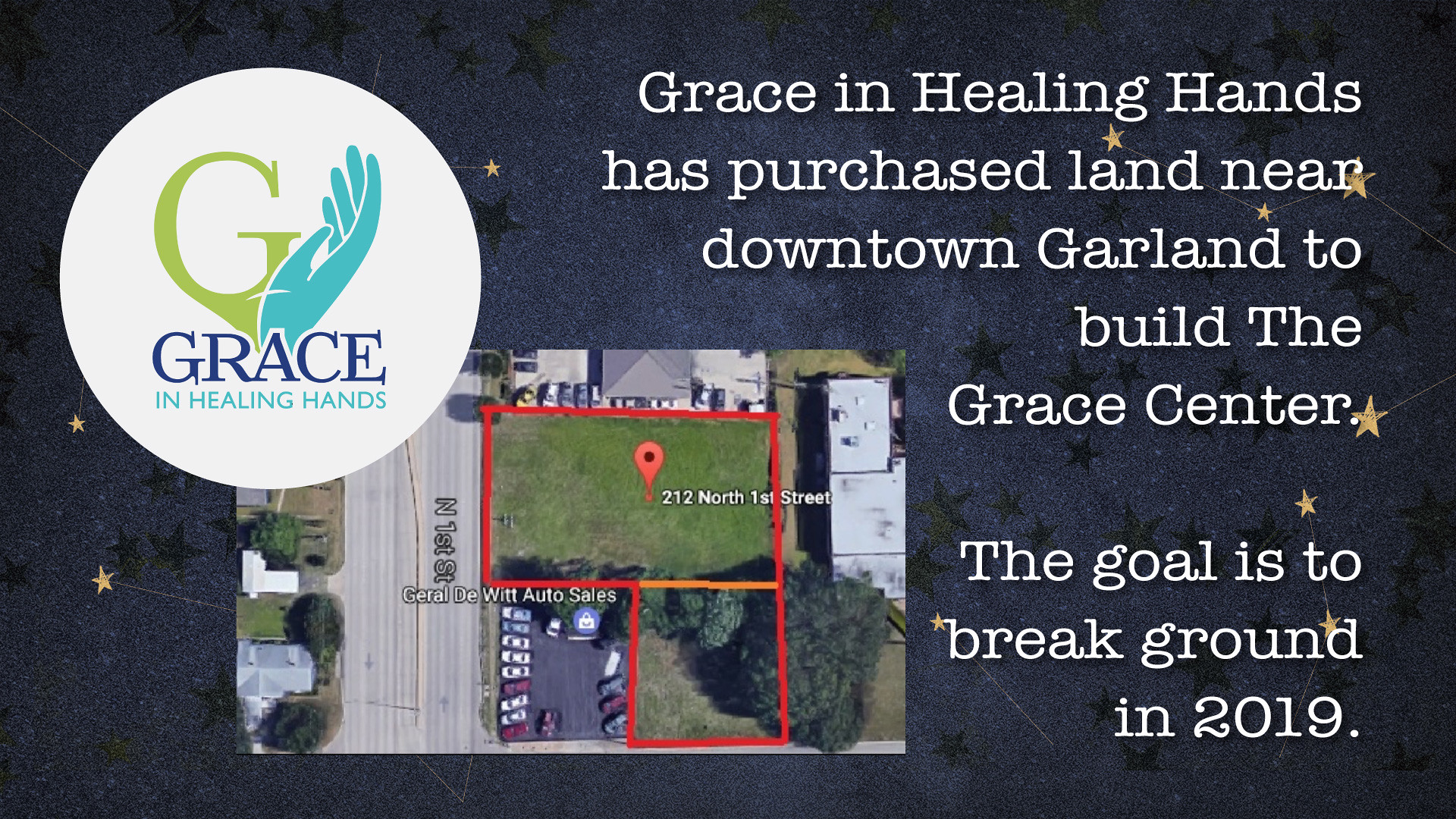The flyer has a dark blue background designed to resemble a night sky, adorned with various black and gold five-point stars. In the upper left corner, a large white circle features a logo with a green letter 'G,' a teal hand, and the words "Grace and Healing Hands" written in blue underneath. Below and to the right of this logo, the flyer includes an aerial, satellite-style photograph showing a plot of land at 212 North 1st Street, bordered by buildings and a parking lot identified as Gerald DeWitt Auto Sales. The plot is currently empty, marked with green space and a few trees. On the right side of the flyer, white text states: "Grace and Healing Hands has purchased land near downtown Garland to build the Grace Center. The goal is to break ground in 2019."